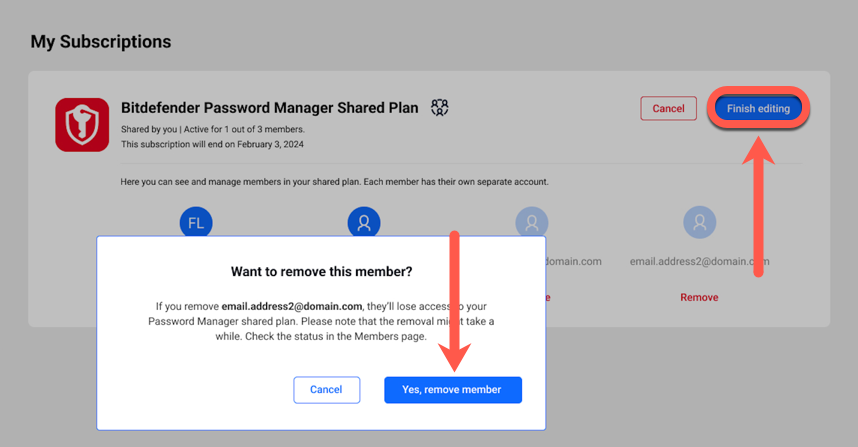The image displays a webpage from Bitdefender's subscription management section. At the top-left corner, the text "My Subscriptions" is prominently shown in black. Below it, details about a "Bitdefender Password Manager Shared Plan" are visible, indicating the plan is shared by the user and is active for 1-3 members. The subscription is set to expire on February 3rd, 2024. Adjacent to the text is the Bitdefender logo, featuring a red square with a key centered in a shield shape.

To the right, there are options to "Cancel" or "Finish Editing," with a blue "Finish Editing" button highlighted by an orange pill-like outline and white text. An orange arrow points upwards towards this button.

In the middle-left section of the screen, the "Manage Members in Your Shared Plan" area is displayed. Each member has their separate account, depicted with circular icons – one with the initials "FL" and others with generic human outlines. Email addresses and domain information accompany these icons.

Towards the bottom-right, there is a removable member section, explaining that if a member is removed from the email address linked to domain.com, they will lose access to the shared password manager plan. It also notes that the removal process may take time and advises checking the status on the members' page. Below this message, there are "Cancel" and "Yes, Remove the Member" buttons, with an orange arrow directing attention to the latter.